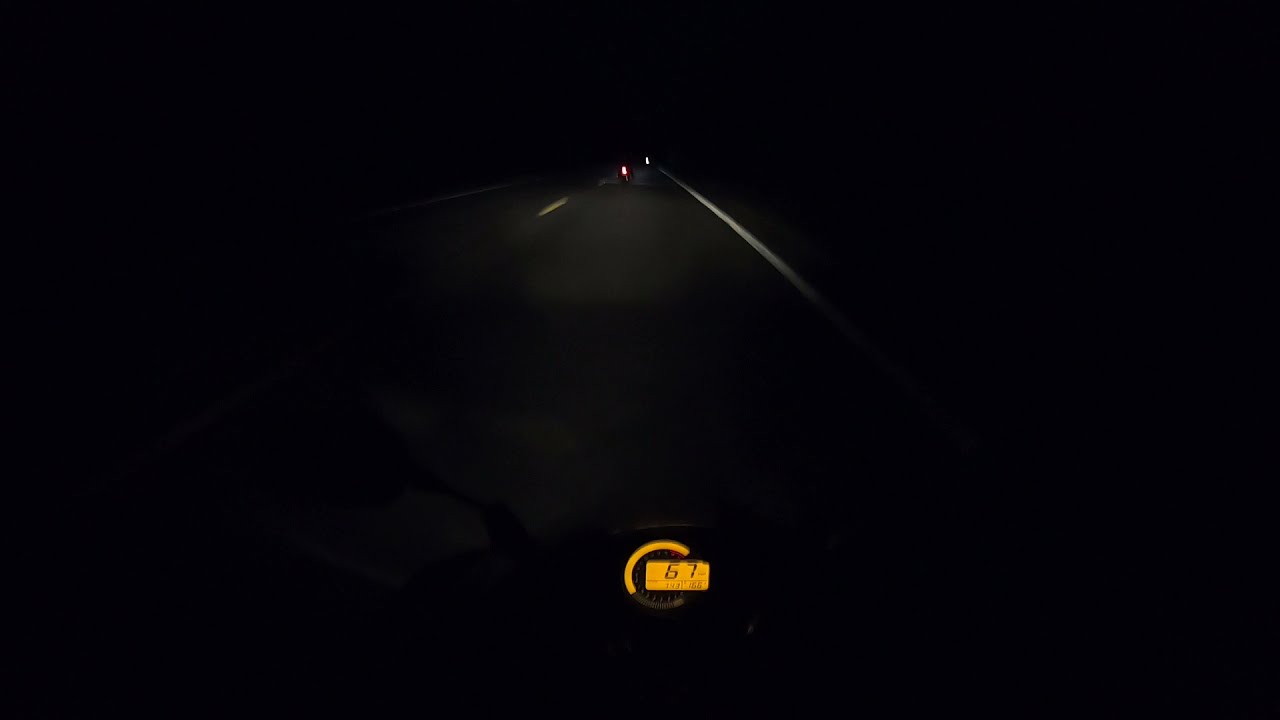In the stark darkness of night, this image captures the intense solitude of a nighttime motorcycle ride. At the center, an orange-lit electronic speedometer glows dimly, marking a speed of 67 miles per hour with black numbers on a golden rectangle display. You can just barely discern the outline of the motorcycle’s front. Ahead, two distant rear lights from fellow riders punctuate the inky blackness. The road, a dark gray asphalt streaked with a dotted white line in the center, runs parallel to a solid white line defining the edge on its right side. The enveloping pitch-black sky and road shoulders enhance the scene's nocturnal intensity and focus on the motorcyclist’s solitary journey.